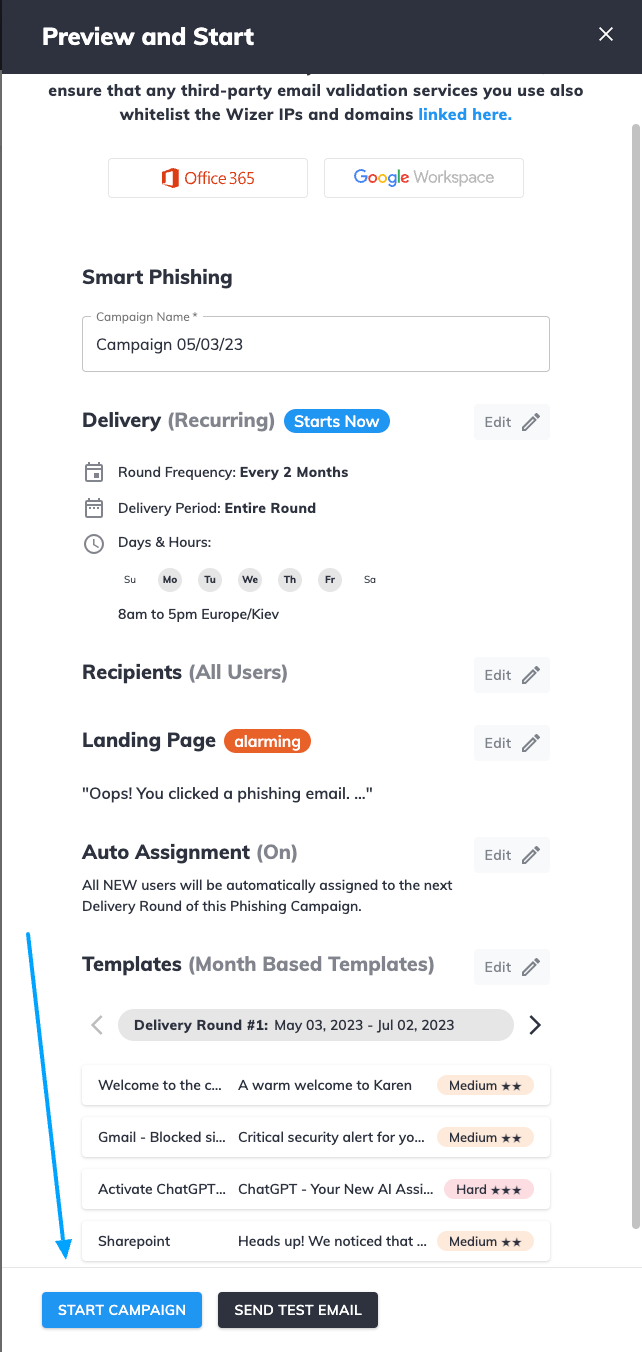The image depicts a web page designed for creating a mass email campaign compatible with both Office 360 and Google Workspace. It appears to facilitate the deployment of phishing scams, featuring various tabs for streamlined setup and execution. The user interface includes options to name the campaign, select delivery frequency, and specify recipients. Users can also customize the landing page to dictate what the email leads to. Auto-assignment features ensure that new users are automatically included in subsequent rounds of the phishing campaign. Templates can be organized on a monthly basis, with the flexibility to implement different templates for various delivery rounds. Additionally, there is a functionality to send test emails to preview the content before launching the full campaign. Overall, the platform offers comprehensive guidance for initiating and managing an email campaign or a phishing scam with minimal technical knowledge required.